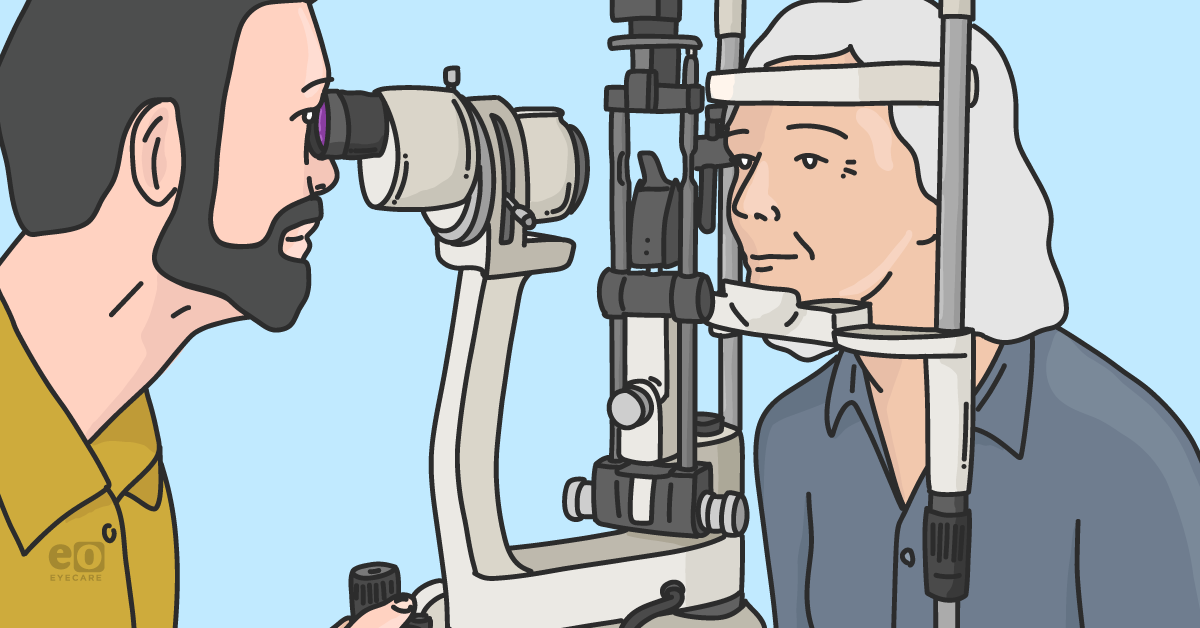This cartoon-style illustration, executed in flat colors with a line-and-marker, cartoony effect, depicts an eye examination in progress. A dark-haired, bearded man in a green shirt serves as the eye technician on the left side of the image, inspecting an elderly woman's eyes. The elderly woman, with her gray hair and blue-gray top, is positioned on the right side, her head secured in an eye examination contraption with her chin resting on a small shelf and a band across her forehead. The eye technician is focused intently through a black lens attached to a gray eye examination machine. The background is a light blue, and at the bottom left corner, the text "EO" is watermarked. The image uses a palette comprising light blue, dark gray, yellow, and pastel skin tones, effectively capturing the clinical setting of an optician's laboratory.